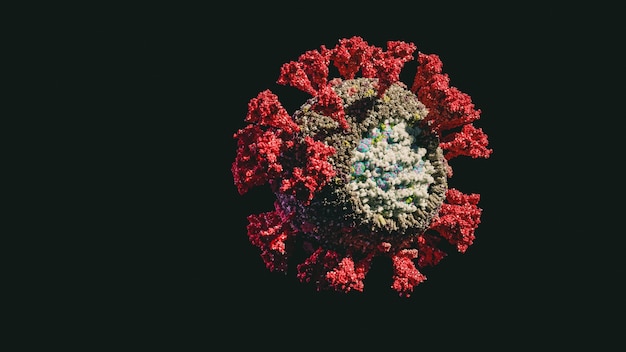The image showcases a 3D render of a virus or viral particle, prominently centered against a completely black background. The central orb-like structure, predominantly dark gray with interspersed lighter yellow particles, features an intricate surface decorated with branching red spikes that resemble tree-like coral structures. These branches are composed of clusters of tiny red balls becoming bushier as they extend outward. At the heart of the orb, there's a pronounced crater filled with larger white orbs surrounded by smaller blue and yellow dots, creating a vivid contrast against the darker base. The red tree-like spikes, combined with the colorful crater elements, contribute to a visually complex and striking depiction.